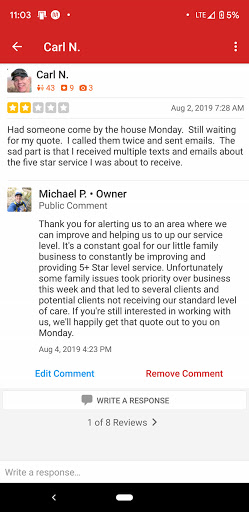The image is a screenshot captured on a smartphone at 11:03, displaying minimal carrier signal and a critically low battery life of just 5%. At the top of the screen, a red notification banner is visible next to a left-arrow icon. The header includes the name "Carl N." accompanied by three white dots on the right. 

In the main portion of the screen, set against a white background, there is a profile picture of Carl N., a smiling man wearing a hat. Carl N.'s profile indicates he has three photos, nine favorite posts, and 43 friends. Below this information, represented by two stars, is a post timestamped at 7:28 AM on August 2, 2019.

Carl N. shares his experience, noting he had someone visit his house on Monday and is still waiting for a quote. Despite his efforts to follow up with calls and emails, he ironically received numerous texts and emails promoting the company's five-star service. In response, Michael P., identified as the owner, appreciates Carl N.'s feedback and assures that the company is committed to improving. Michael P. expresses the company's ongoing dedication to striving for five-plus-star service, underscoring their commitment to continual improvement in their small family business.